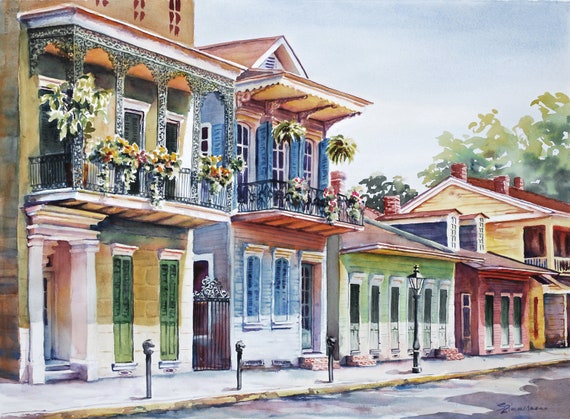This is a painting resembling an idyllic row of historic townhouses, invoking the vibrant architecture often seen in New Orleans. The series of structures is closely arranged, with some potentially connected and others suggesting narrow alleyways between them. The painting is done in a detailed, painterly watercolor style utilizing pastel colors that bring a soft yet colorful ambiance to the scene.

At the far left, the first townhouse, painted in greens, is distinguished by its sizable two-story facade, featuring a large balcony shaded with greenery, Romanesque columns framing the entrance, and two long, skinny windows on the lower level. Adjacent to it, the second building is a light blue two-story structure, mirroring the previous one with its balcony and plants on the upper level. Progressing to the right, the buildings transition to single-story structures, with the third being in green, followed by a red-colored building. The sequence culminates in another double-level structure painted in yellow, where only a part of the upper balcony is visible.

The scene is set against a white and blue sky with trees peeking from the background, emphasizing the vibrant and lively yet quaint atmosphere. The painting includes street elements like a sidewalk, a road running parallel to the row of houses, old-fashioned street lamps, parking meters, and the artist's signature discreetly placed in the bottom right-hand corner.